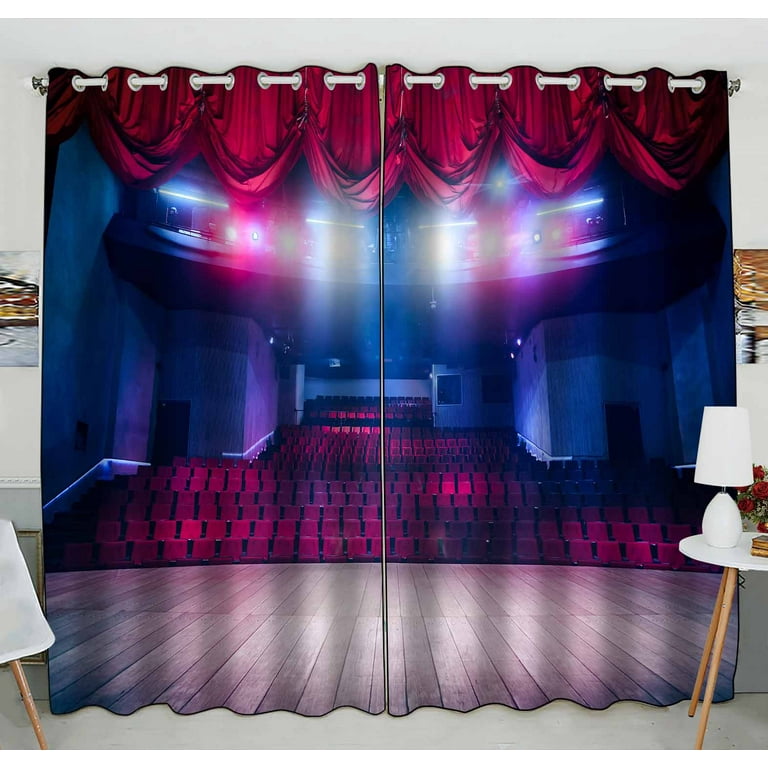This detailed colored photograph captures a theatrical stage setting, but intriguingly, it is an image of an intricately designed curtain that portrays a stage and an audience. The curtain is split into two parts and hangs from a white rod with silver ends and white circular hooks. The curtain itself features an image of an empty theater, showing a wooden stage floor and rows of red seats beneath stage lights.

On either side of the curtain, the room's walls are white with two pictures displayed, one picture with shades of grey, black, brown, silver, and tan hangs on the left side, and the other, incorporating brown, beige, and white, is on the right. At the bottom left corner, there is a table with brown wooden legs and a white tabletop, holding a white lamp with a white lampshade. On the right side, another table with similar wooden legs and a white top supports a white lamp, a book with yellow and green cover, and a bouquet of red flowers with white accents and green stems.

The floor of the room is grey, while the baseboard running along the walls is white. Above the curtain, lights in the ceiling shine red and blue, enhancing the theatrical ambiance of the scene. Despite the detailed imagery on the curtain, the illusion of a stage and audience adds to the photograph's depth and complexity.